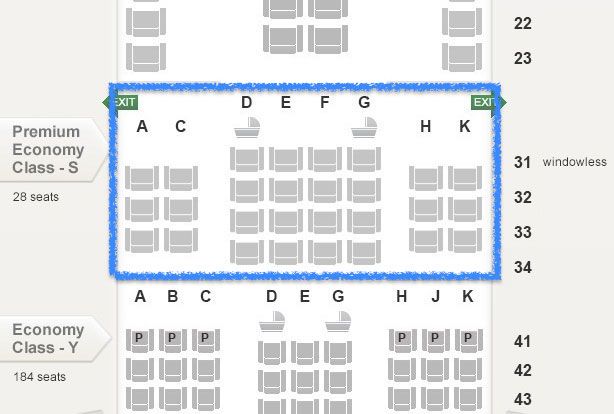The image depicts a detailed seating plan for an airplane. The background is a light gray, contrasting with the darker gray icons representing individual seats, viewed from a top-down perspective. Within this layout, most seats are oriented to face straight ahead, but notably, four specific seats are angled to face the left.

At the top of the image, two seats are positioned one above the other. In the middle section, there's a row of two adjacent seats. To the right, a vertical pair of seats is arranged, one directly behind the other. 

A distinct square section highlighted in blue is centrally located in the seating arrangement, corresponding to rows A, C, D, E, F, G, H, and K. To the left side of this blue-highlighted area, there is a section denoted as premium economy class (S), followed by the broader economy class (Y).